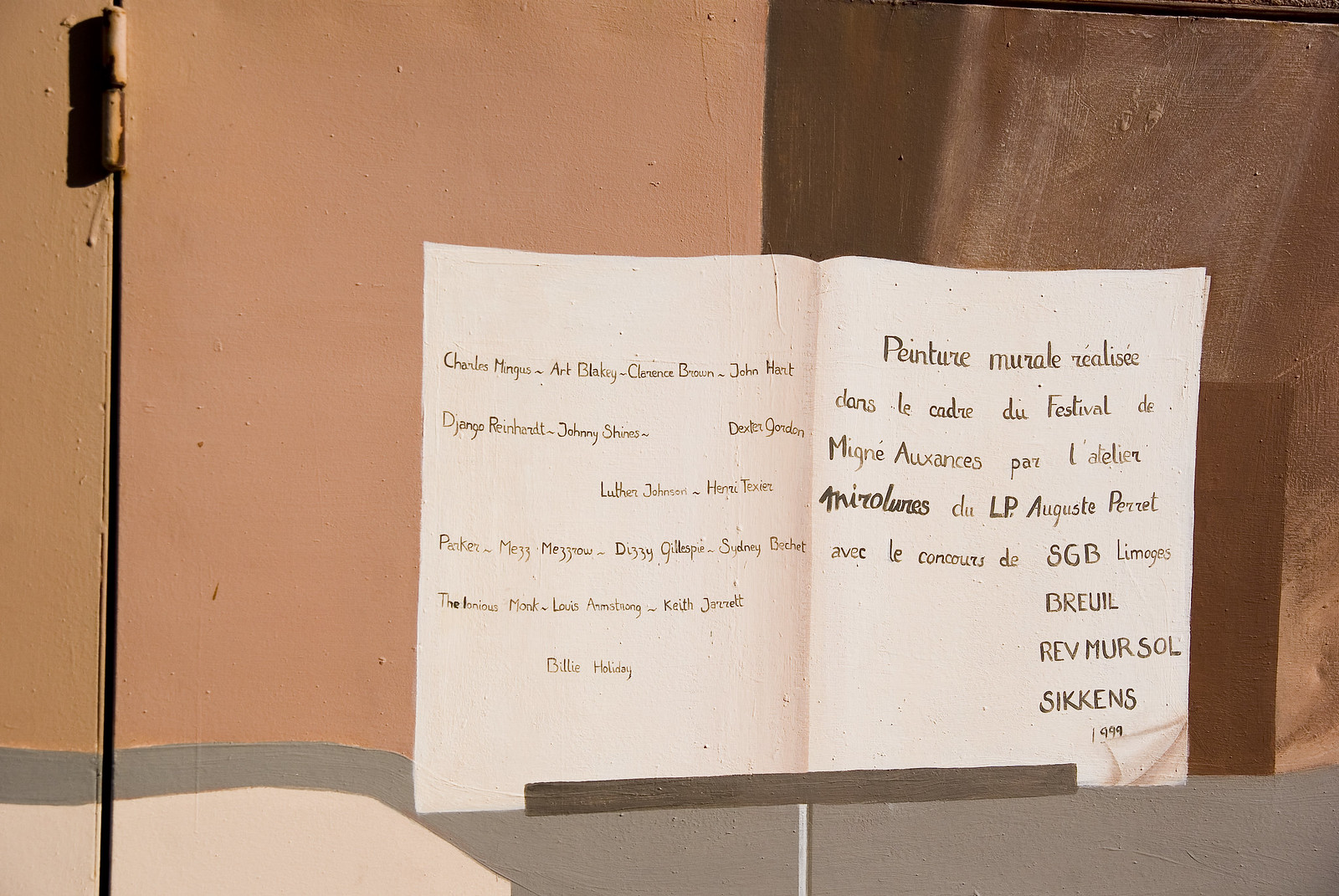The image depicts a detailed mural with a multi-colored background wall featuring a tan left section, a brown right section, a gray bottom section, and a pale peach lower left corner. Central to the mural are two painted pieces of paper. The left page lists names of prominent jazz musicians such as Charles Mingus, Art Blaski, Clarence Barron, John Hart, Django Reinhardt, Johnny Shins, Dexter Gordon, Luther Johnson, Dizzy Gillespie, Keith Jarrett, Billie Holiday, Louis Armstrong, and Thelonious Monk Parker. The other page contains text in an unfamiliar language. The mural's design resembles the folding pages of a book, and it is marked with the year 1999 on the bottom right corner.